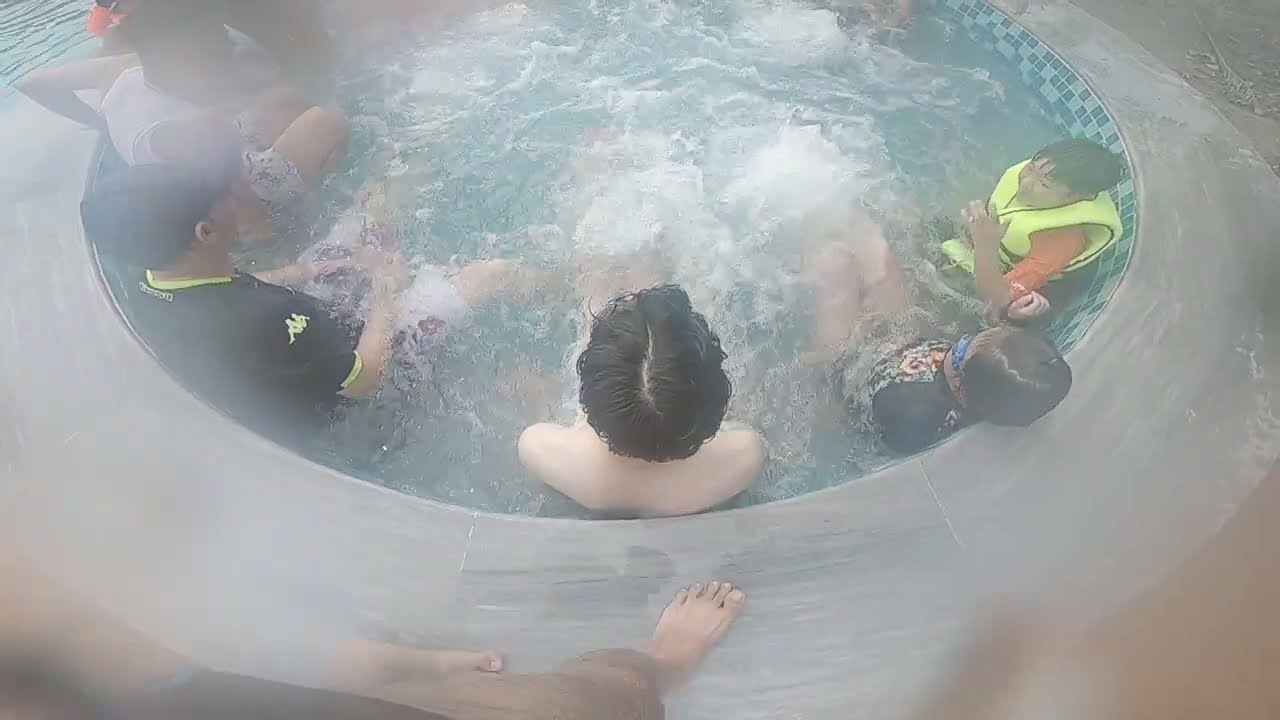In this overhead shot of a hot tub, the camera captures a scene where various people are seated and enjoying the bubbling water, giving the viewer a top-down perspective. The presence of water droplets on the camera screen adds a hazy effect, making some details appear slightly blurry. The hot tub itself is adorned with tiles of different shades of light and dark blue, while the surrounding area is paved with concrete.

On the far right, there's a young boy distinguished by his bright yellow life jacket and red shirt. Beside him, a person in a black top sits close. Next to them, a shirtless man with black hair faces away from the camera. Further left, another man, attired in a black shirt and matching black hat, is visible. Additionally, you can spot a person in a white sleeveless top and printed shorts, although they appear somewhat blurry.

The image also shows frothy, churning water, indicative of the vigorous jets typical of a hot tub. At the very bottom center of the image, there is the partial view of a person's legs and foot, likely someone standing just outside the hot tub on the concrete edge. Overall, the hot tub scene is a vibrant mix of colors and textures, framed by the lively motion of the water and the varied attire of the people immersed in it.